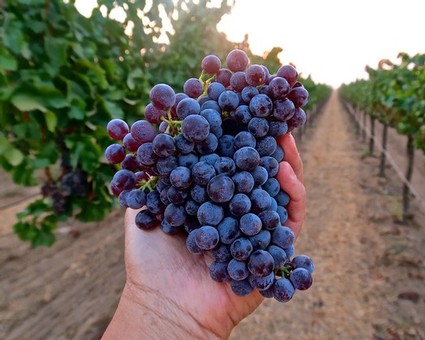In this vibrant vineyard scene, an individual holds up a large, freshly-picked cluster of purple grapes, showcasing their glossy and healthy appearance. The person's left hand firmly grasps the clump, displaying the grapes, which vary in hue from light to dark purple. The hand obscures whether it belongs to a man or a woman. The backdrop reveals rows of grapevines stretching into the distance, possibly several hundred yards, bordered by rows of meticulously maintained vines on both sides of a dirt path. The vineyard is well-organized, with vines held upright by white ropes ensuring orderly rows. The soil is visible between the rows, illustrating the cultivation setting. Though the sky is slightly blurred, the focus remains on the ripe, enticing grapes. This thriving vineyard could be situated in a renowned wine region such as Europe or California, though the exact location remains undefined.